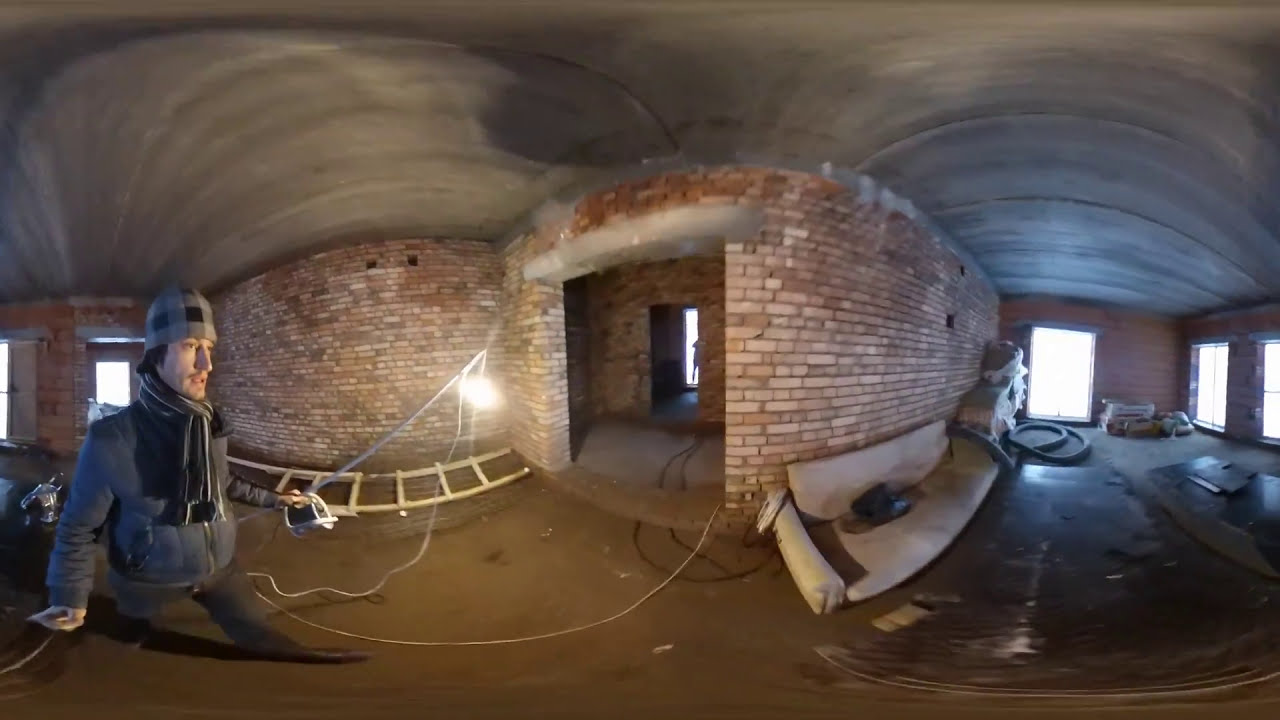The image depicts an indoor setting, likely an unfinished building or underground parking structure, characterized by its curved, cavernous form. The floor appears to be unfinished concrete, and the brick walls feature several openings suggesting ongoing construction. The ceiling, resembling cement with horizontal brush stroke designs, further adds to the raw, industrial feel of the space.

On the left-hand side, a man in a gray jacket and a gray and black plaid hat walks, illuminating the brick wall with a light in his hand, creating a focal point in the scene. He also wears a scarf around his neck. The distorted view makes his legs appear stretched and elongated, reminiscent of a Funhaus mirror effect.

Nearby, a light tan ladder lies on its side in the middle left of the image. On the right side, half of a couch is visible with a green bag resting on it. Above this, two circular, possibly green objects are seen in the upper part of the image. The building features windows allowing natural light to filter in, heightening the sense of an unfinished, industrial workspace.